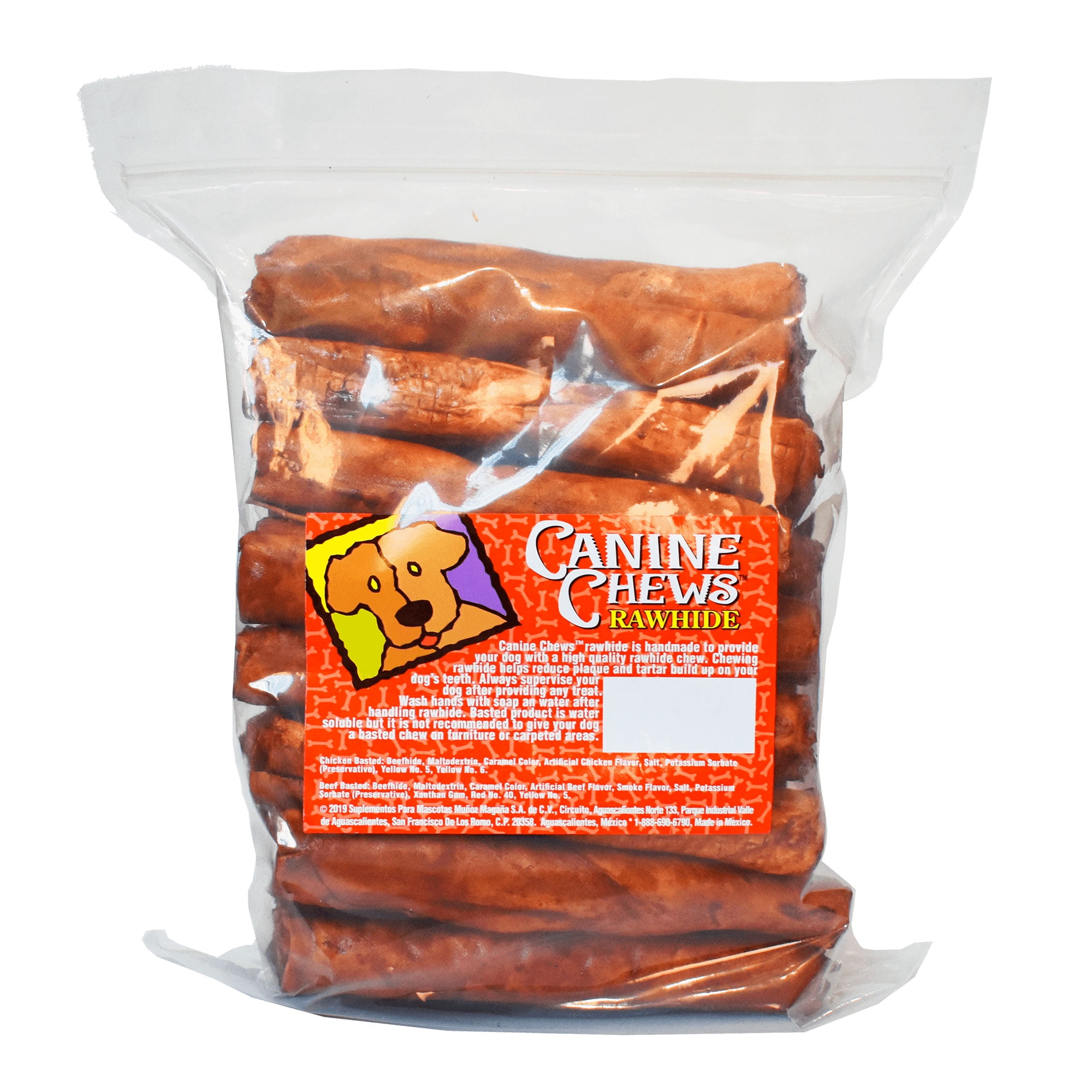The image shows a clear plastic bag filled with approximately a dozen brownish-reddish rectangular rawhide canine chews, stacked horizontally from left to right. The packaging prominently features a red label in the center, adorned with numerous small white bone motifs. On the upper left corner of the label, there is an abstract illustration of a tan dog with yellow eyes, a black nose, and a red tongue sticking out, set against a background split into yellow and purple panels. The text on the label includes "canine chews" in white and "rawhide" in yellow, along with small, hard-to-read white text likely describing the product.